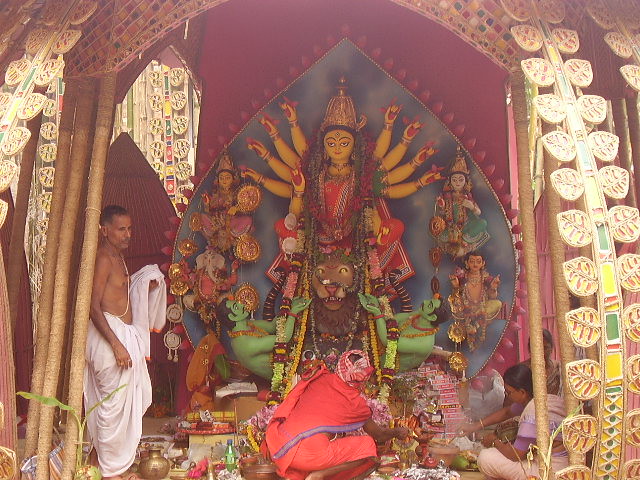The vibrant outdoor daytime scene captures a Hindu religious shrine adorned with intricate, colorful decorations featuring maroon, yellow, pink, white, and gold accents. The central focal point is an elaborate statue of a goddess with eight arms, adorned with beads and surrounded by smaller deities. The statue is situated against a purple backdrop and is flanked by multicolored elements including flowers and green statuettes.

In the lower right corner, a man stands dressed in a white sheet wrapped around his lower body, his upper body bare. Nearby, a woman clad in purple is kneeling as she lights incense. Centrally, another man dressed in red with a turban sits cross-legged, leaning to his right and seemingly in prayer or deep contemplation.

Next to the central statue, multiple subjects engage in various acts of devotion: some kneeling, others sitting in the classic Indian-style pose, all fixated on the goddess statue. The rich tapestry of colors and the detailed arrangement of the shrine, complemented by the devotees' reverence, evoke a profound sense of spirituality and cultural heritage.